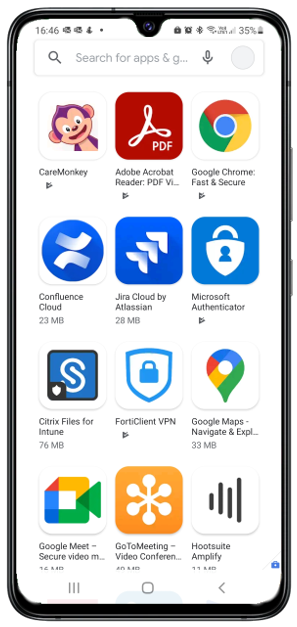This image is a screenshot of a smartphone's home screen displaying a variety of applications. The first app in view is "Care Monkey," which is represented by an icon featuring a cartoon monkey. Following that is "Adobe Acrobat Reader" with the familiar Adobe icon, known for its red and white color scheme. The "Chrome" app icon is also present, displaying its characteristic colorful wheel. "Confluence Cloud" is included with an icon depicting a cloud, signifying its cloud-based functionalities. 

Additionally, "Microsoft Authenticator" is among the apps, typically used for secure sign-ins, though its icon is not described in the screenshot. "Google Maps Navigation" is present as well, known for its detailed maps and directions services. The "Port Client VPN" app is shown, usually providing secure remote network access. 

The list continues with "Google Meet," used for secure video conferencing, marked by its camera icon, and "GoToMeeting," another video conferencing tool, but its icon isn't specifically detailed in the screenshot. "HootSuite Amplified" is another app available, represented by its distinctive owl icon, known for managing social media accounts. "Cloud Files" appears next, most likely for cloud storage, but its specific icon is not detailed.

At the top of the homescreen, there's a search bar equipped with a microphone icon, indicating voice search capability. Lastly, the app "GyroCloud" is visible, with an icon showing a blue box featuring three white arrows, possibly signifying data transfer or movement within a cloud service.

The overall arrangement of these apps suggests a focus on productivity, communication, and cloud-based services, tailored for both personal and professional use.